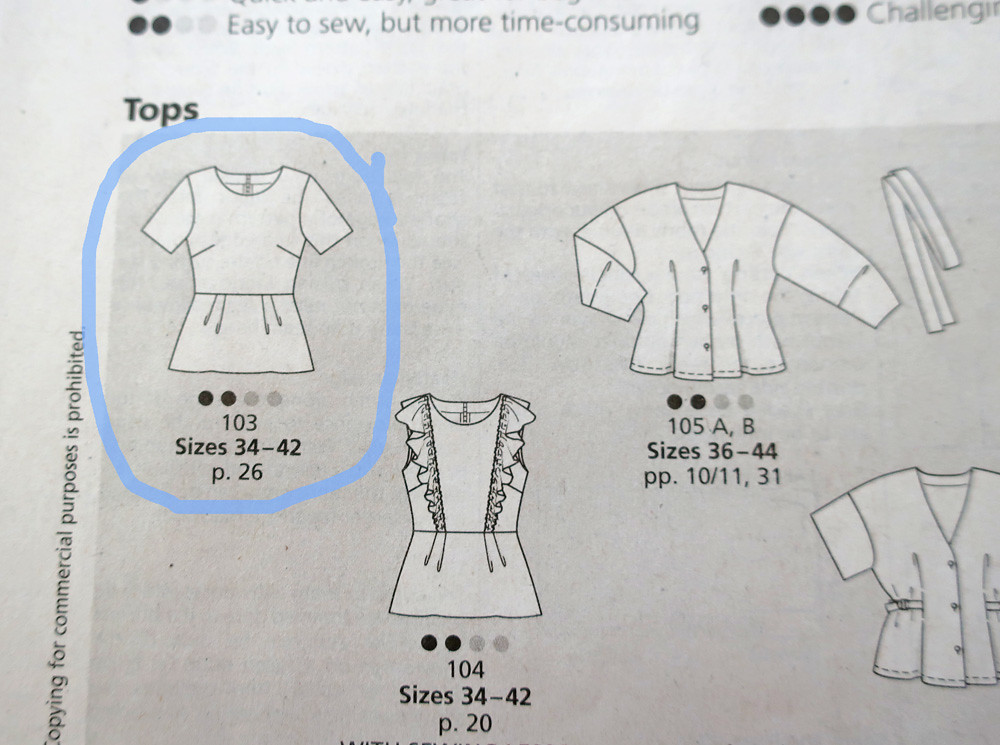The image depicts an up-close photograph of a sewing pattern instruction sheet. The background is a white-gray color, and the top of the page is cut off. At the top of the image, in black text, it reads "easy to sew but more time-consuming" with two of four circles filled in black, and to the right, partially cut off, it says "challenging" with all four circles filled. Below this, there is a section headed by the word "tops" in black text over a darker colored box.

Within the darker box are several illustrated diagrams of various clothing tops. The first top on the left is an outline circled in blue. Below it, the text indicates "103 sizes 34 to 42" and continues with "P26". The next top to the right is a long-sleeve garment labeled "105 AB sizes 36 to 44" and includes additional text "pp 10/11 31". Below these, aligned beneath the first top, is a sleeveless top with ruffles, annotated with "104 sizes 34 to 42 page 20". To the right of this top, partially cut off at the bottom and right edge of the image, there appears to be a short-sleeve shirt that is buttoned down the front and belted.

Along the left edge of the darker box, vertically aligned text states "copying for commercial purposes is prohibited," with the "C" in "copying" cut off at the bottom of the image. The detailed diagrams provide numbers and sizing information for each top, and the partially visible elements hint at additional contents beyond the current frame of the photograph.